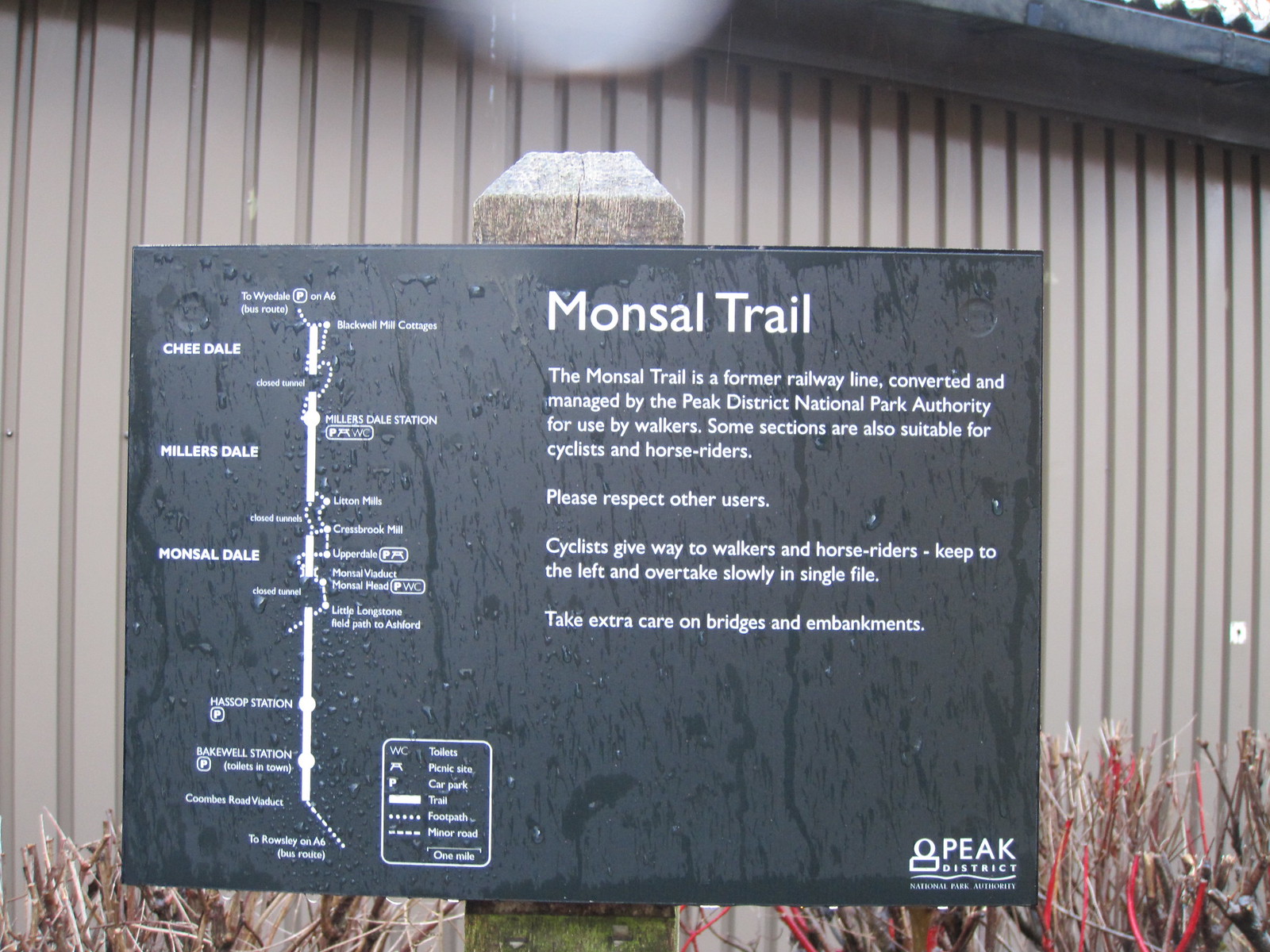This image shows an outdoor information board displaying details about the Monsal Trail, positioned near a beige-colored building. The sign is mounted on a wooden post and features a black background with white text. At the top, it reads "Monsal Trail." Below, it explains that the Monsal Trail is a former railway line converted and managed by the Peak District National Park Authority for use by walkers, with some sections also suitable for cyclists and horse riders. The sign advises users to respect others: cyclists should give way to walkers, horse riders should keep to the left and overtake slowly in single file, and caution is urged on bridges and embankments. On the left side of the sign, there is a map of the trail with various explanations, and in the bottom right corner, there's a logo for the Peak District National Park Authority. At the base of the sign, some bare brown branches or sticks are visible.